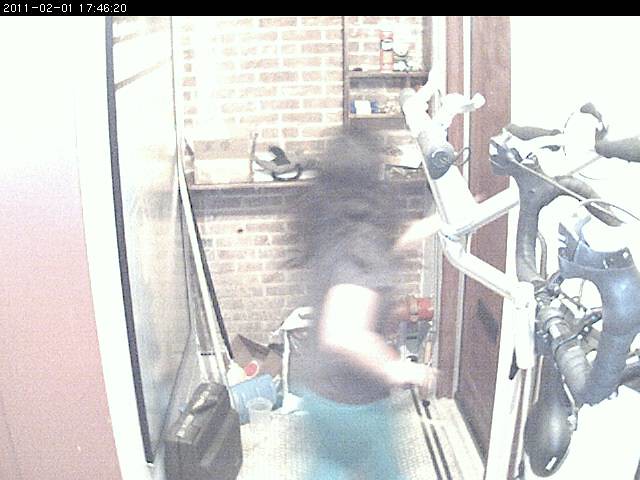A rectangular screen capture from a camera showcases an individual adjusting exercise equipment. The image features a black banner along the top edge, stretching from the top left to the top right, displaying a timestamp in white text: "2011-02-01 17:46:20". In the center of the frame stands a person with long dark hair, dressed in a short-sleeved brown shirt and blue pants. They are seen touching the white frame of the exercise equipment, which is securely mounted on a white wall. The scene takes place in a small, narrow room with a tan carpet featuring black stripes along its sides.